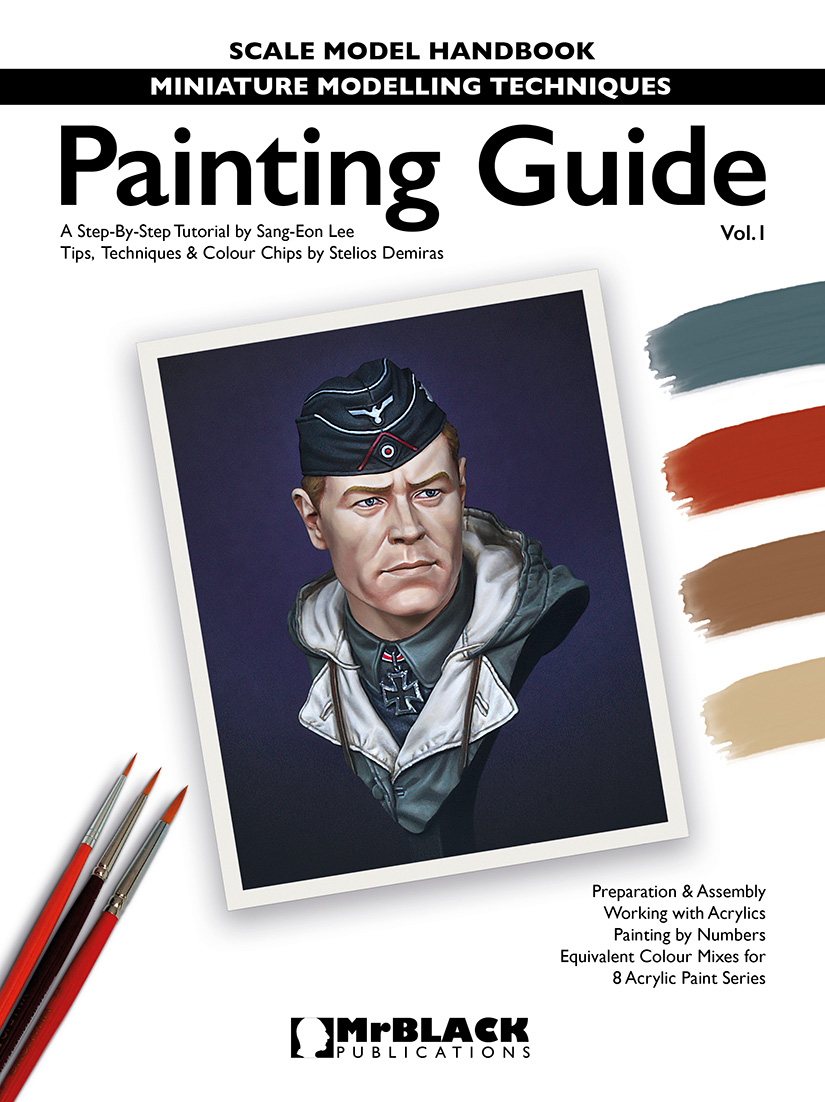This image is the cover of "Scale Model Handbook: Miniature Modeling Techniques - Painting Guide Volume 1" by Mr. Black Publications. At the top, "Scale Model Handbook" is displayed in prominent black block text. Below it, within a thin black stripe, "Miniature Modeling Techniques" is written in white lettering. Larger black text below this reads "Painting Guide." In smaller black text beneath "Painting Guide," it states, "A Step-by-Step Tutorial by Sang-Ian Lee," followed by "Tips, Techniques, and Color Chips by Stelios Demirez.” Under the 'E' of "Guide" is the subtitle "Volume One" in very small black text.

The center features a stylized photograph with drop shadows on a navy blue background that transitions from dark corners to a lighter center. The image depicts a middle-aged Caucasian soldier, his bust showing a uniform that suggests a German military affiliation. He has blonde hair, chiseled features, and is wearing a military cap adorned with an iron eagle, accompanied by a hooded jacket and an iron cross at the collar.

On the lower left side of the cover, three paintbrushes are depicted; two are red with metal caps and one is black with a red tip. To the right, four painted strips represent paint swatches in gunmetal blue, carmine red, brown, and taupe beige hues. 

At the bottom center of the cover, the Mr. Black Publications logo is displayed. In the lower right, five lines of small black text list the contents: "Preparation and Assembly," "Working with Acrylics," "Painting by Numbers," "Equivalent Color Mixes for Eight Acrylic Paint Series."